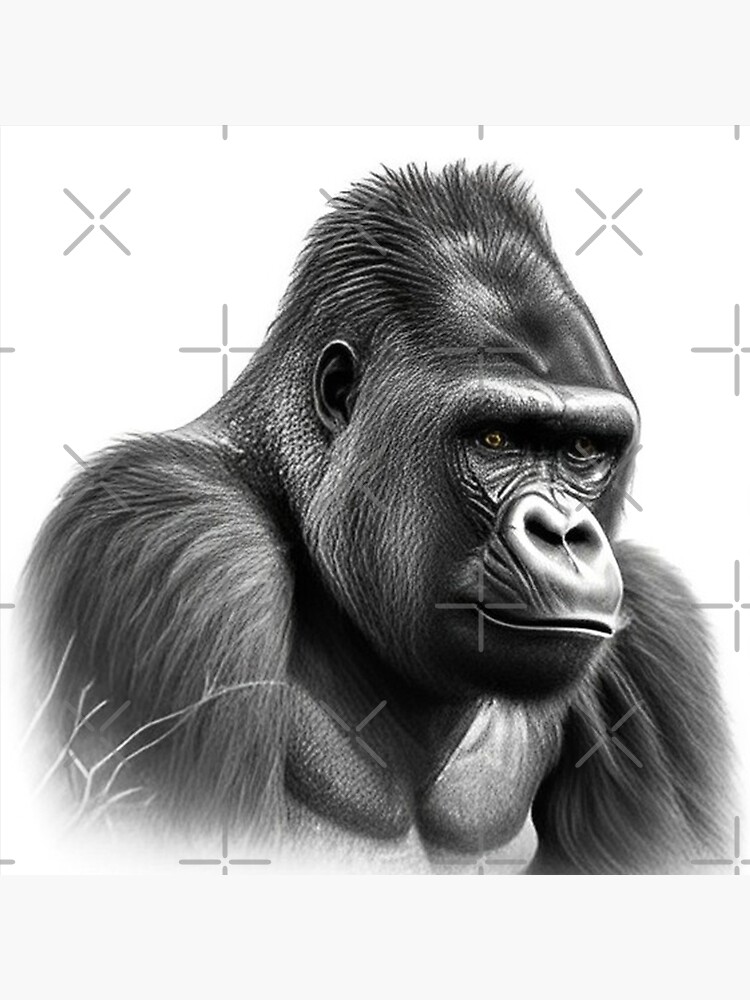This is a highly detailed, black and white drawing of a gorilla, skillfully rendered using pencil or charcoal. The composition captures the head, upper chest, and shoulders of the gorilla against a stark white background adorned with abstract gray X's and crosses, adding texture and depth to the image. The gorilla, occupying three-quarters of the image space, is depicted with meticulous attention to detail—the individual hairs on its head and fur are finely illustrated. The gorilla's expression, which could be interpreted as contemplative or frustrated, features small eyes that slightly suggest a hint of brown, although the piece is primarily monochromatic. Its mouth is closed, and the animal is gazing to the right, adding a sense of stillness and introspection to the artwork. The overall effect is enhanced by the intricate shading and highlights, creating a lifelike representation that almost appears illuminated by an unseen light source.